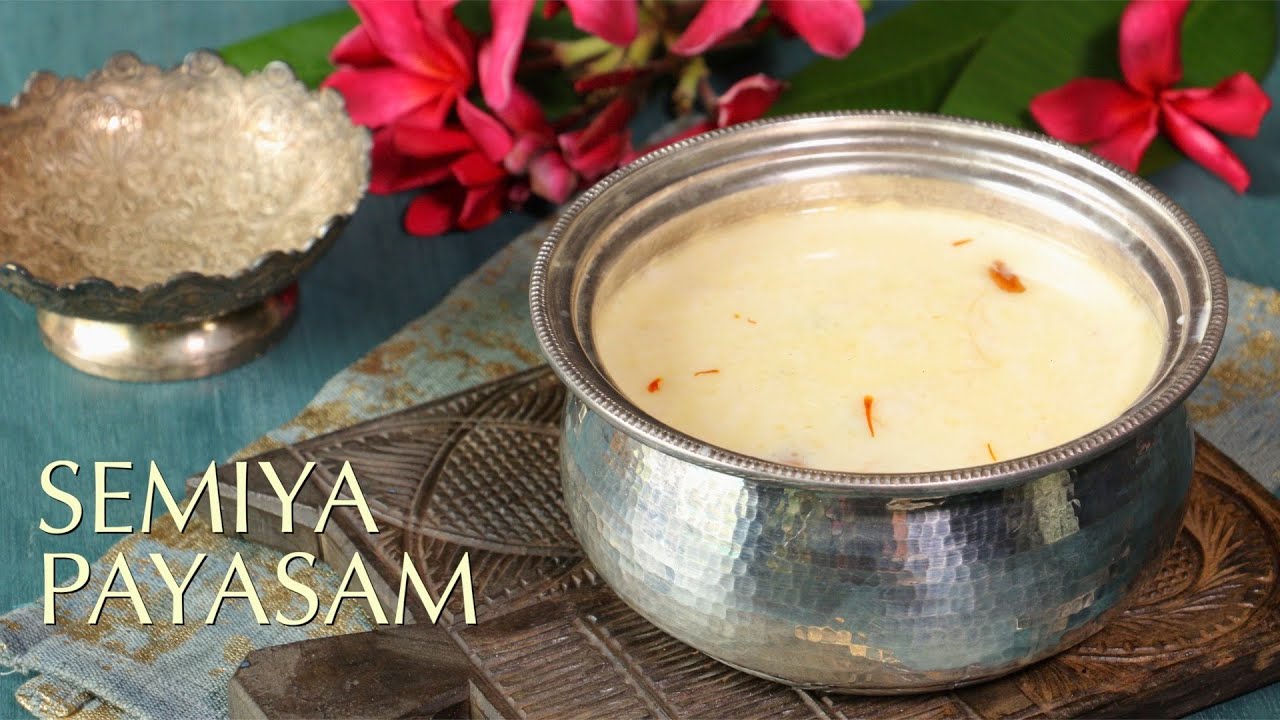The image features a polished silver bowl or pot, intricately designed with indents, containing a pale beige or off-white colored soup with red or orange flecks, suggesting it might be a creamy potato or vegetable-based soup. The pot is set on a stone trivet atop a table. Surrounding the pot are decorative elements: a small container that could hold rings or jewelry, and vibrant red flowers adding a splash of color to the scene. The table also bears an inscription in tan writing, "Semia Payasam," indicating the name of the dish, which is a traditional Indian dessert. The photo is horizontal, capturing these elements in detail and creating a warm, inviting culinary setting.